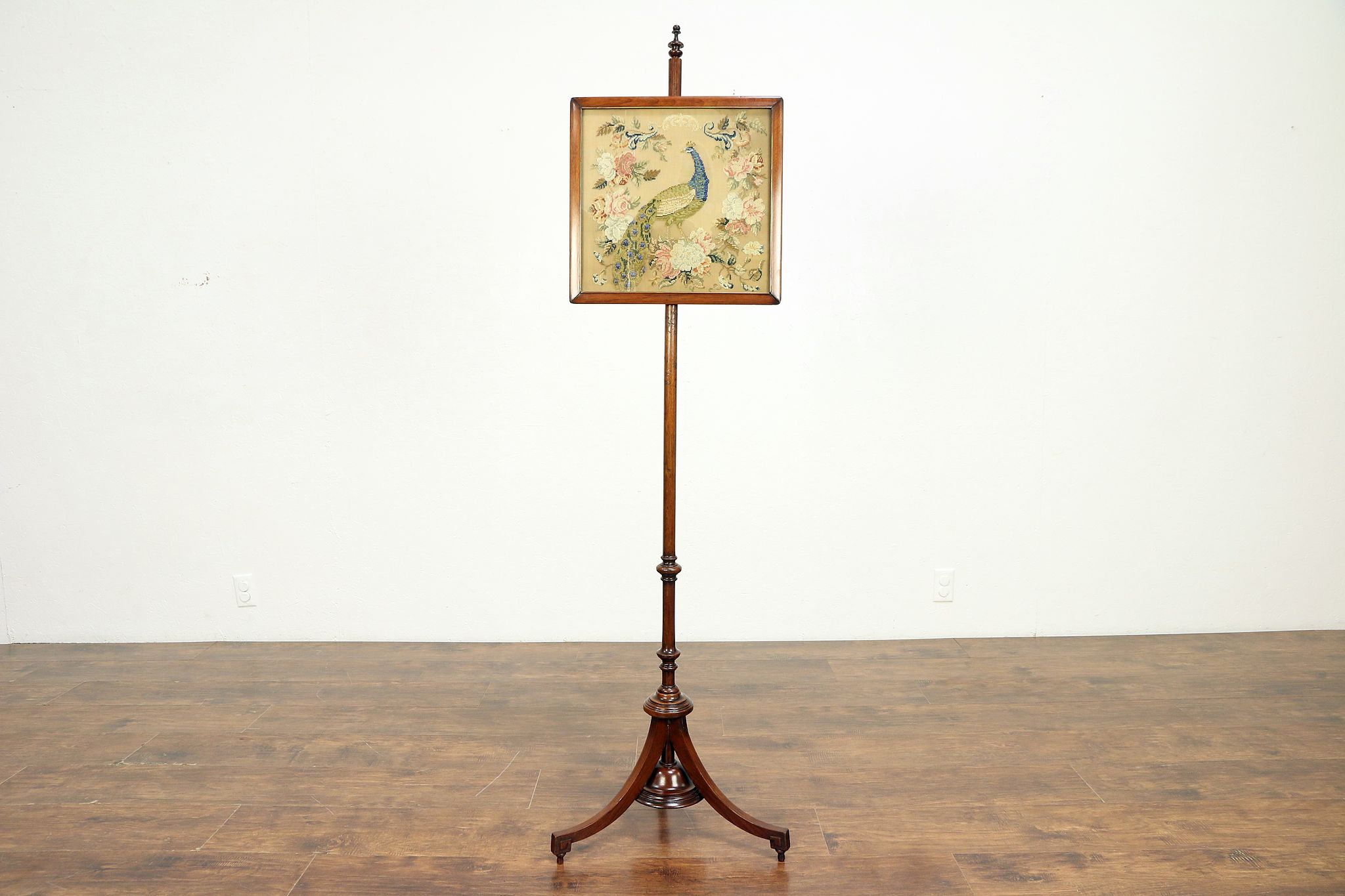The image captures a rectangular photograph of a minimalistic room featuring a stark, off-white wall and an aged, yet well-maintained wooden floor exhibiting brown and black hues. Central to the composition is an elegant wooden stand, characterized by its thin, stained pole and tripod base. This stand supports a square wooden picture frame that beautifully matches the pedestal's wood tone. Framed within is a detailed depiction of a male peacock, rendered either as a painting or needlepoint, showing off its elaborate tail adorned with various elements. The peacock boasts a striking blue head and neck, with the rest of its plumage in shades of beige and yellowish tones. The artwork's background is predominantly tan, accentuated by a fanciful U-shaped border composed of white and pink flowers. The room is largely unembellished, directing full attention to the exquisite centerpiece.